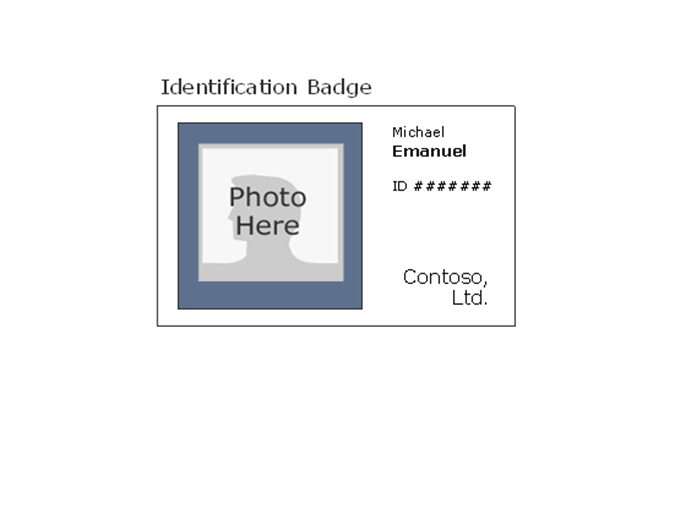The image displays an identification badge, rectangular in shape with a length shorter than its width. At the top of the badge, the words "Identification Badge" are printed in black. On the left side, there’s a blue photo frame containing a photo of a human face, shoulders, and legs, with the phrase "photo here" overlaid. The badge has a light gray shape with a white background. On the right side, the name "Michael Emmanuel" is printed, with "Emmanuel" in bold. Below the name, an ID number is listed, followed by seven numerical digits. At the bottom of the badge, it is branded with "Contoso Ltd."